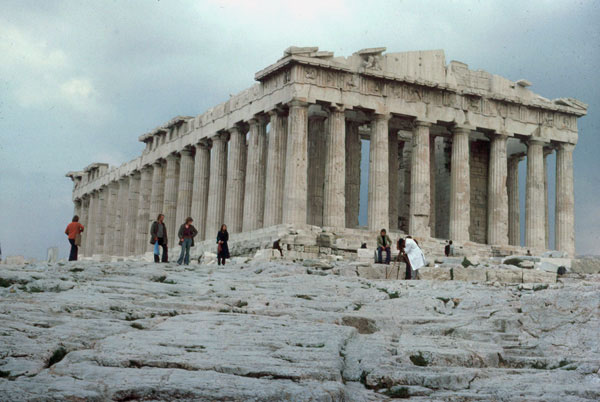The photograph captures an ancient rectangular temple-like structure, reminiscent of Greek architecture, with remarkable marble columns adorning its perimeter. The once-grand roof is now mostly crumbled and missing, revealing the dark, cloudy gray sky above. Positioned on a rocky elevation, the ruins convey a sense of monumental history. The scene is outdoors during the day, with a group of people scattered around the foreground of the ruins. Their attire is notably from a bygone era, featuring black and blue bell-bottoms paired with orange, brown, and tan jackets, indicating a dated fashion style from a few decades back. Among the visitors, a person on the right stands out in a white doctor's coat, another lounges in a tan business suit with denim jeans while seated on a square rock. Meanwhile, three individuals—two women and a man—appear to be students, engaging with the person in the white coat. Despite the ominous sky hinting at possible rain, the historical site and its visitors clad in warm clothing suggest an intriguing juxtaposition of the ancient past with mid-to-late 20th-century nostalgia.